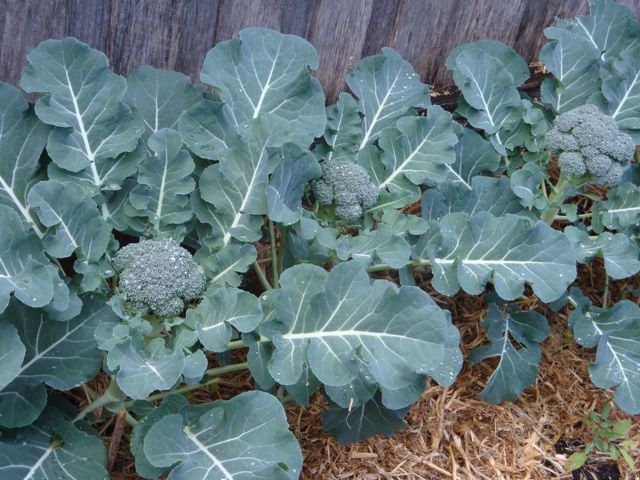This color photograph, taken in landscape orientation, depicts an outdoor scene featuring three large heads of broccoli positioned side-by-side near the base of an old, smoky gray picket fence that runs horizontally across the top of the image. The broccoli heads are surrounded by lush, scallop-shaped leaves in a dark, bluish-green hue with prominent yellowish-white veins. The leaves create a dense canopy, almost completely enveloping the bushy, green florets of the broccoli. Below the canopy of leaves, the ground is covered with a layer of straw-like tan mulch that has a slight golden-yellow tint, with a noticeable patch of brown grass interspersed with green plant edges in the bottom right corner of the photograph. The detailed textures and contrasts create a rich and dynamic composition, highlighting the earthy, natural elements of a garden setting.